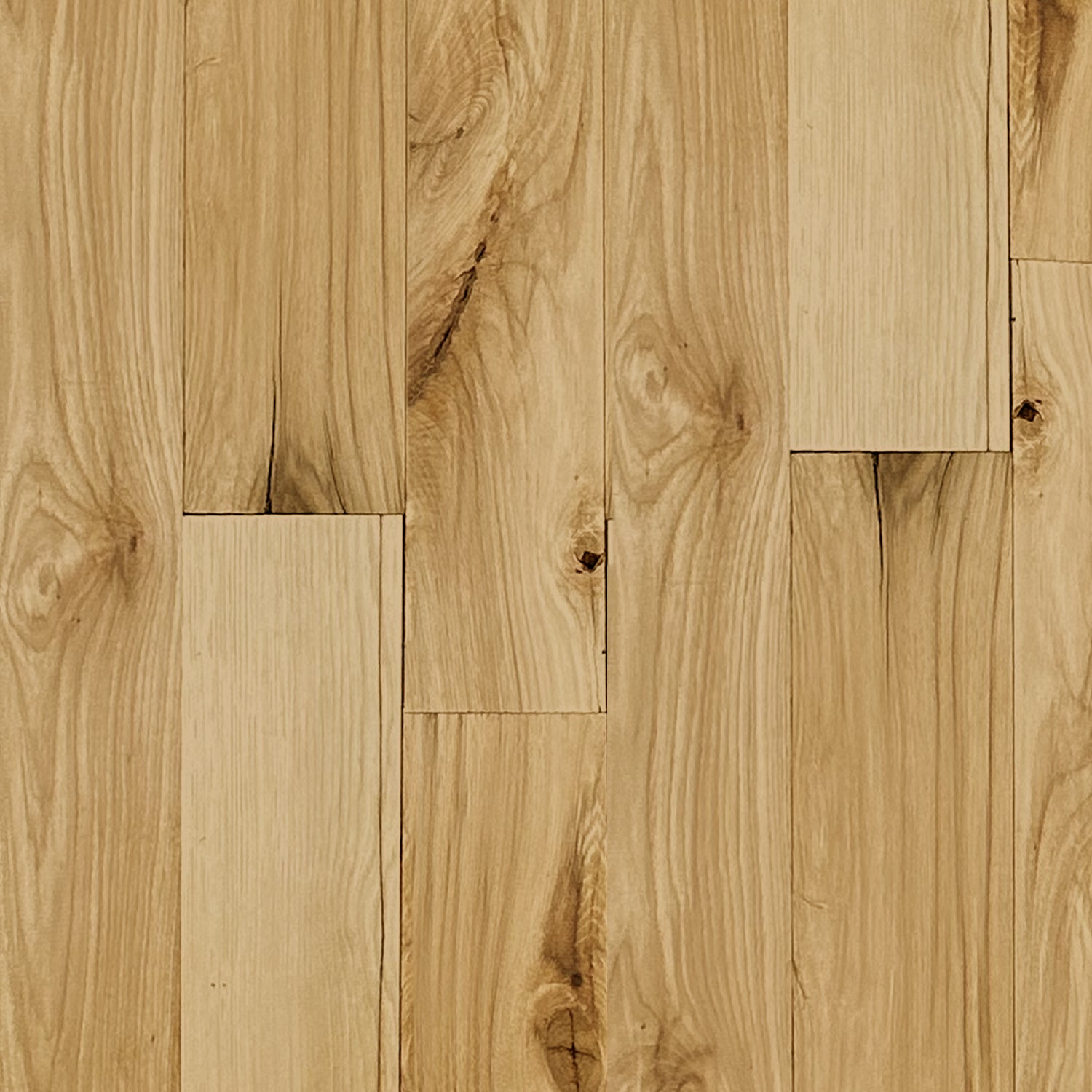This square image depicts a segment of a rustic wooden plank floor, characterized by its light-colored, natural wood appearance. The planks exhibit an array of imperfections, including small black holes, darker brown knots, and various streaks, contributing to the floor's unique character. Each plank is distinct, with some appearing lighter and smoother while others are darker and more textured. The arrangement of the planks is not uniform, featuring alternating solid and paired planks that create a patchwork effect. The detailed patterns where the wood pieces come together, along with the visible joints and natural blemishes, emphasize the authentic, unfinished look of the wood. Overall, the flooring has the visual depth and variation reminiscent of luxury vinyl tiles designed to emulate real wood.